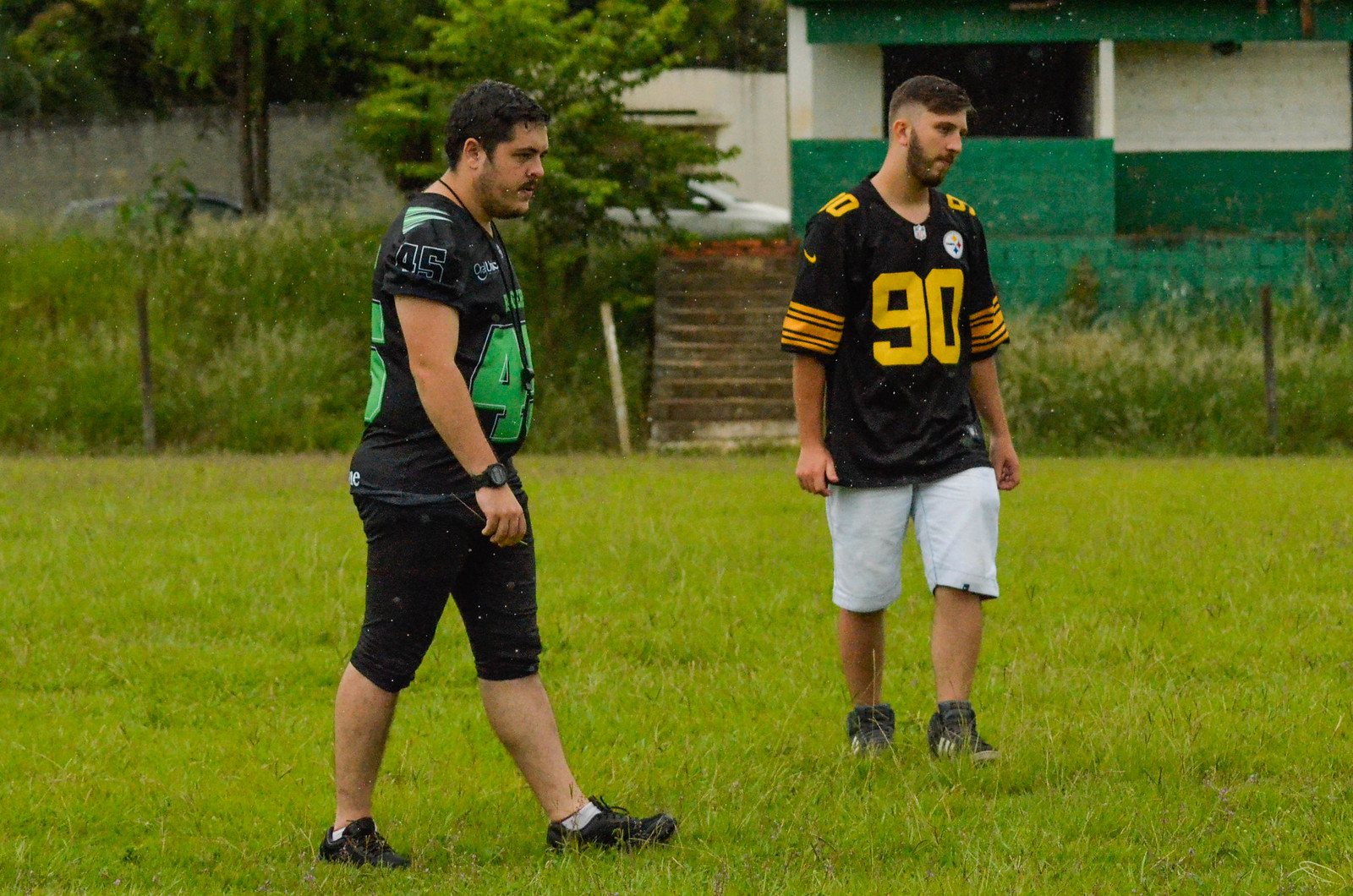In the image, two white men with beards are captured in mid-motion on a grassy field. The man on the left has dark curly hair and is wearing a black jersey with green numbers, paired with short pants, and black Adidas cleats. He appears to be walking forward, his second foot just starting to lift off. Beside him, the other man sports short black hair and a beard. He is dressed in a black jersey with gold numbers and similar shorts, also wearing black cleats. Both men are looking towards the right. The grass they are walking on is a bright lime green, interspersed with some taller weeds. In the background, a mix of bushes and a tree can be seen along with a green and white building and brown steps, likely indicating some sort of exterior facility. There are also hints of cars and perhaps another brick structure. The overall setting suggests an overcast but daylight atmosphere.